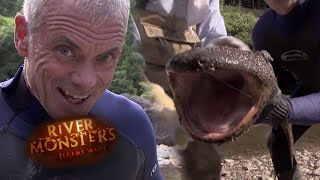The image is a promotional screenshot for the TV show "River Monsters." On the left side of the photo stands the show's host, an older Caucasian man with short, white hair and blue eyes, dressed in a blue wetsuit. He is smiling deviously at the camera. The show's logo, "River Monsters," displayed in gold letters on a brown background, is positioned close to his chin. To the right of him, a giant eel-like creature is being held by another person, who is also dressed in a wetsuit with gloves and long sleeves. The creature, which resembles a gigantic salamander, is brown in color, has visible eyes, and its mouth is wide open, revealing a pink interior. Behind them, faint greenery can be seen, adding a natural backdrop to the scene. The overall setup suggests a thrilling encounter with the bizarre and creepy creatures featured in the show.